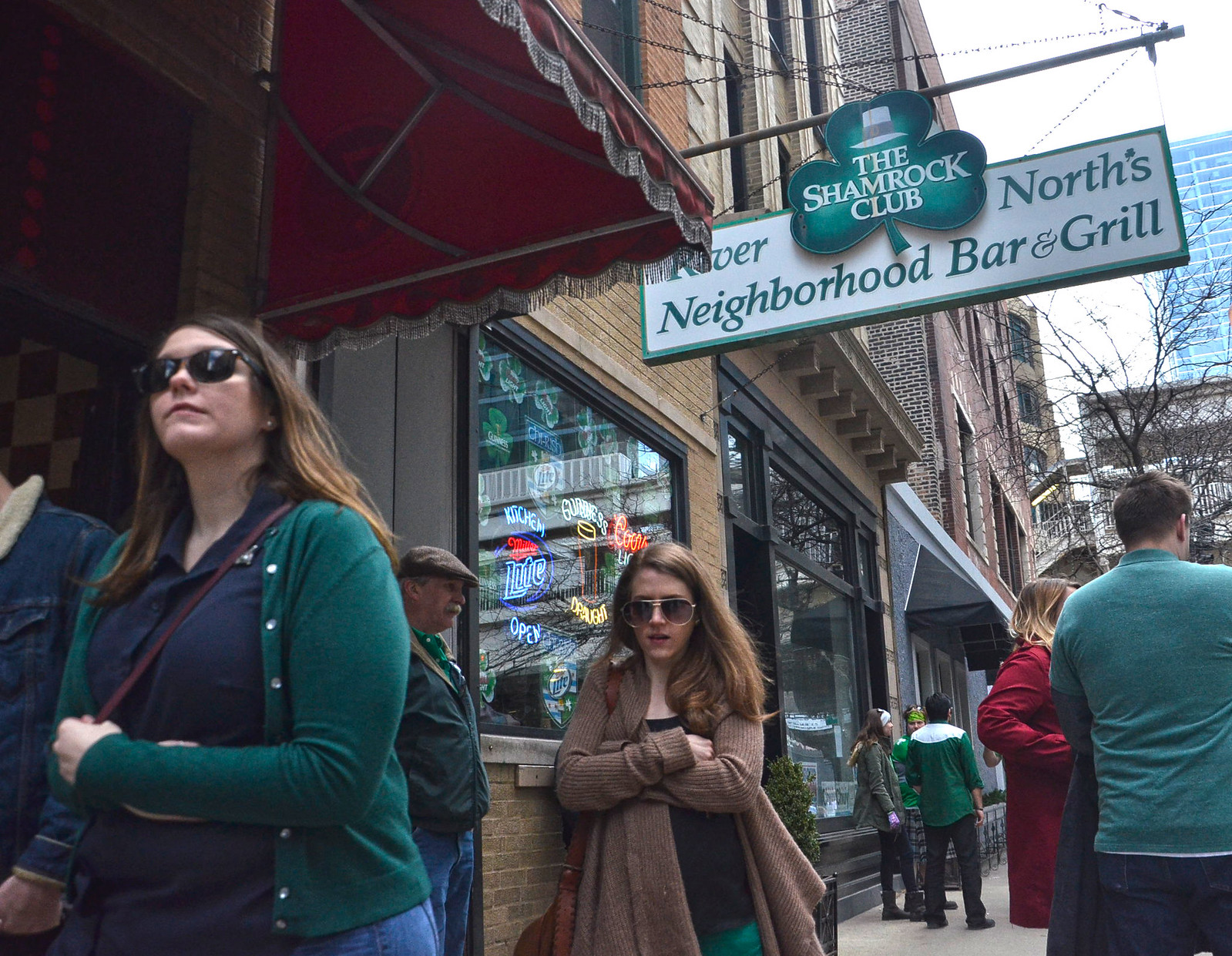The photograph captures a lively scene outside an establishment called The Shamrock Club, River North's neighborhood bar and grill, on St. Patrick's Day. Dominating the upper part of the image is a large sign with a clover at the center, announcing the bar's name. A bustling sidewalk stretches in front of the bar, lined with various shops. A red awning is adjacent to the sign, and to the right stands a large office building with numerous windows.

The crowd is evidently celebrating, with many of the people donning green attire. In the foreground, a woman with a blue shirt and green sweater has her purse slung across her body and wears sunglasses. Near her, another woman in green leans against the wall. A young lady in a red trench coat-like jacket stands somewhat obscured on the right, while another passerby wears a brown sweater with a black top paired with green pants. The animated scene epitomizes St. Patrick's Day festivities in a bustling downtown neighborhood.